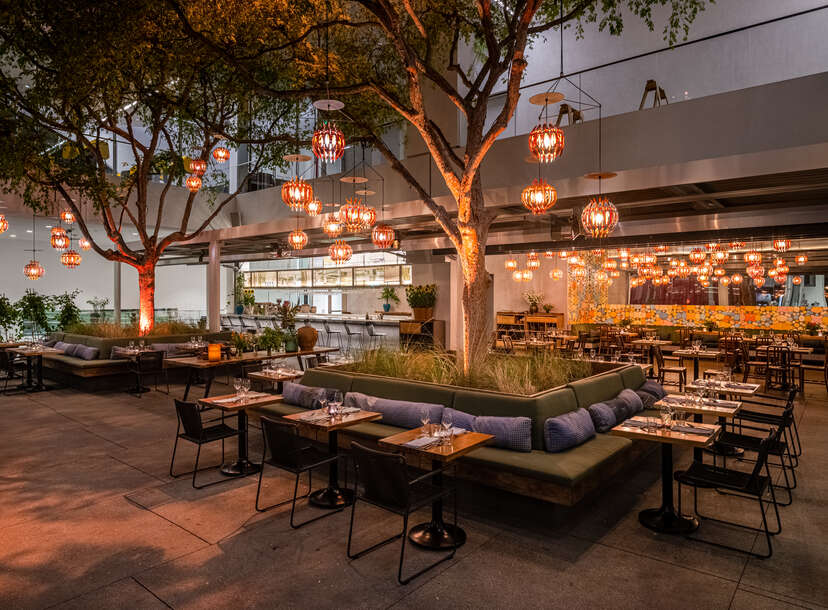The image depicts a modern and stylish outdoor dining area, likely part of a restaurant. Central to the image is a tree encircled by a green upholstered sofa lined with blue cushions, providing a cozy seating arrangement for diners. Surrounding the tree are several square tables set with glasses and napkins, ready to serve guests. The dining area features additional rectangular planters filled with tall green grasses and more trees.

The restaurant itself is a sleek concrete structure with two levels, characterized by its rectangular shape. The upper level, separated by a see-through balcony railing, contains various unidentified items, possibly step ladders. The ground level opens up to the outdoor seating area equipped with brown square tables and black chairs that complement the cushioned benches. Orange and yellow lanterns hang from the branches of the tall, leafy trees, enhancing the ambiance with a warm glow. Similar lanterns are also visible inside the building, suggesting a consistent decorative theme throughout the premises.

In the background, the exterior of the building is marked by the name "Olympia 2," visible on a black awning, with an inviting display of open windows and door frames, hinting at the modern interior dining space that echoes the chic outdoor setup.